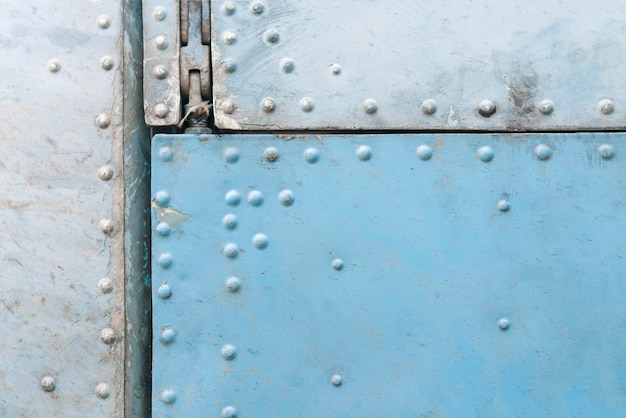The detailed, descriptive caption combining the key points from all three voice descriptions:

The image is a full-color photograph taken outdoors under natural light, depicting a series of metal plates assembled together closely, without any visible borders or background. Prominently featured is a gray metal plate on the left side, adorned with a central row of rivets running vertically along its right edge. This gray piece connects at the top to another smaller gray panel, which is further characterized by horizontal lines of rivets. Dominating the upper portion of the composition is a horizontally rectangular light gray panel, extending towards the right. Below this, a blue panel occupies the lower right section, punctuated by numerous rivets. The colors in the image include shades of light blue, light gray, black, and white. The metal surfaces appear smudged and weathered, suggesting age and wear, and the raised rivets give the impression of textured, bumpy markings. These rivets, scattered across the panels, might carry a hidden meaning, perhaps akin to braille, although their purpose isn't immediately clear. Overall, the arrangement and the signs of wear suggest a functional, yet antiquated metal door.